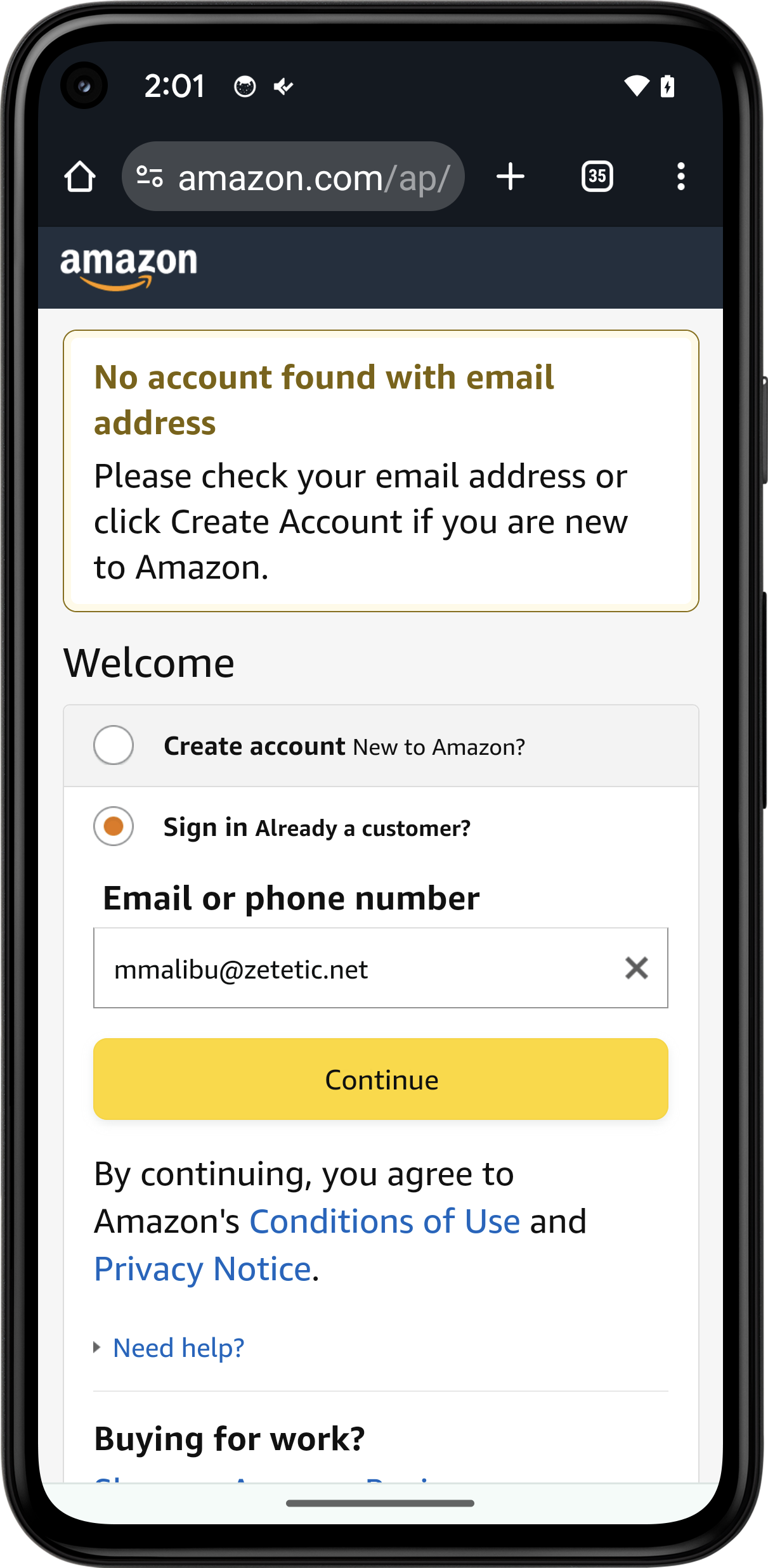The image displays a mobile phone screen showcasing the sign-in page of Amazon's app. The top segment of the phone screen indicates it is 12:20 PM, with active Wi-Fi and a charging battery icon visible. In the upper right corner, there are two unidentified icons. 

The primary focal point is the Amazon login interface where the user appears to be attempting to sign in. A conspicuous red box at the center of the screen alerts the user with the message: "There was a problem." Below this, in black text, it states, "We cannot find an account with that e-mail address." The email address entered is MikeMalibu@zetetic.net.

Beneath this error message, an orange "Continue" button is prominently displayed. In smaller black text below the button, the terms "By continuing, you agree to Amazon's" are followed by hyperlinked terms "Conditions of Use" and "Privacy Notice" in blue. Additional help options like "Need help?" are listed further down.

At the very bottom of the screen, in a less prominent section, are links to "Conditions of Use," "Privacy Notice," and "Interest-Based Ads." The legal footer notes "© 1996-2020, Amazon.com, Inc. or its affiliates."